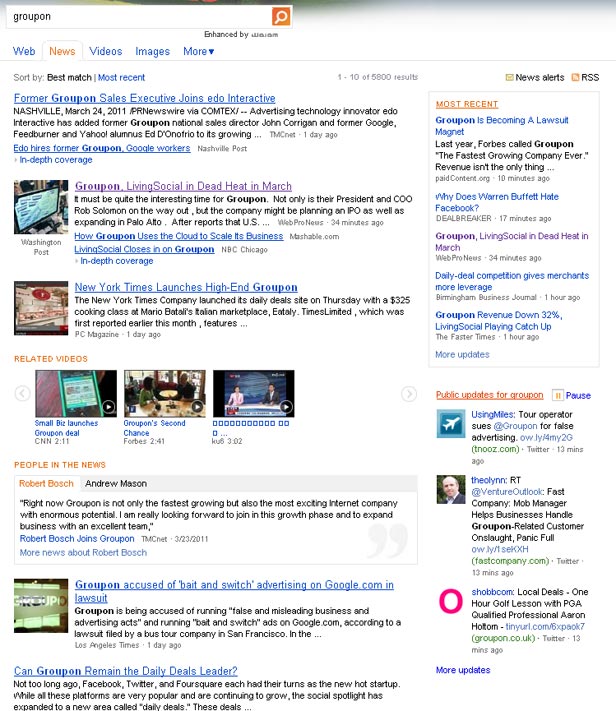The image depicts a search engine results page focused on the term "Groupon" entered into the top search bar. To the right of the search bar, there is an orange square with a magnifying glass icon inside. Below the search bar are various search options including "Web," "News," "Video," "Images," and "More." The "News" option is highlighted in orange text.

Several results are visible on the page:
1. The first result, highlighted in purple text with an underline, is titled "Former Groupon Sales Executive Joins Edo Interactive."
2. Another headline in purple text, also underlined, states "Groupon, Living Social in Dead Heat in March."
3. A blue-underlined link is titled, "New York Times Launches High-End Groupon."

In the center of the page are images, including a cell phone and newscasters sitting at a table. The right side of the page prominently features a news section. Here, the most recent headline reads, "Groupon is Becoming a Lawsuit Magnet," presented in purple text. A duplicate of the earlier headline "Groupon, Living Social in Dead Heat in March" also appears in purple text.

Additional links include:
- "Public Updates for Groupon," highlighted and underlined in orange text.
- An image of a white airplane within a blue square accompanies the link titled, "Tour Operator Sues for False Advertising."
- There is also an image of a bald man in a suit.

Finally, the last visible headline reads, "Venture Outlook: Fast Company Mob Manager Helps Businesses Handle Groupon-Related Customer Onsite Panic."